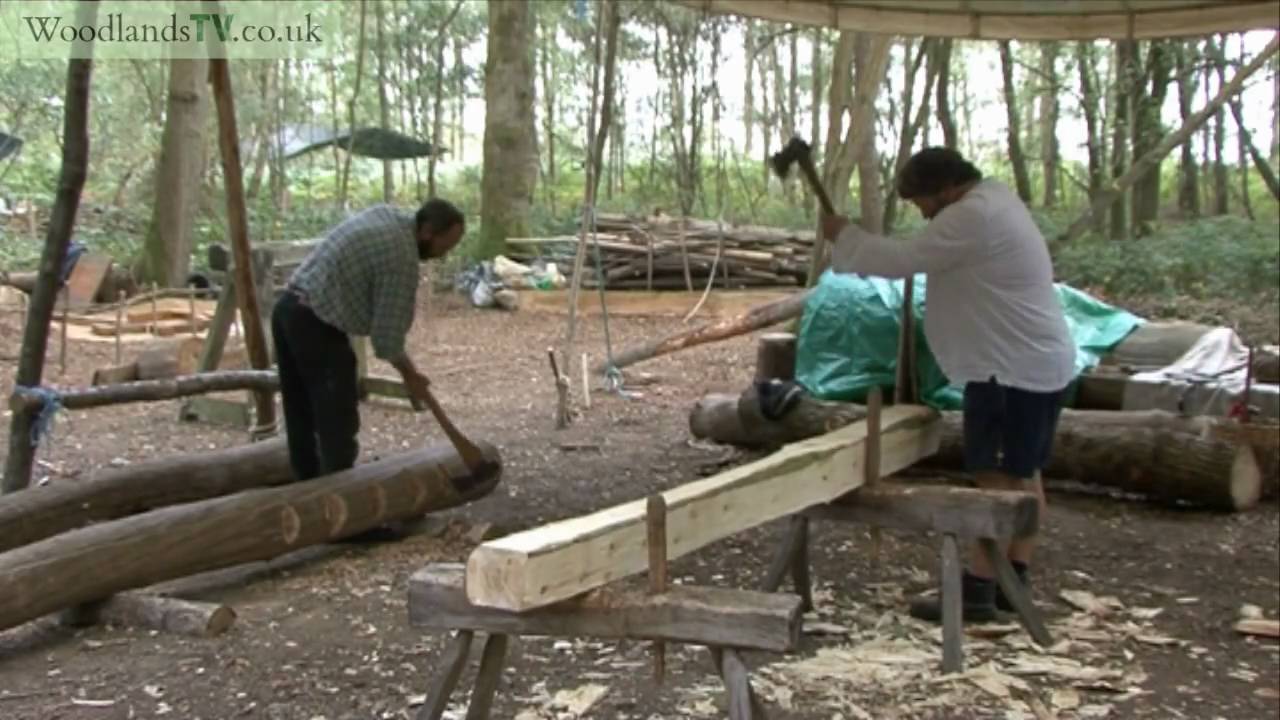In this outdoor, amateurish and slightly blurry image, the upper left corner prominently displays the watermark "woodlandstv.co.uk." Set in a woodland area with abundant brown logs and green foliage, two men, both appearing to be in their 40s or 50s with dark hair and goatees, are focused on chopping wood. The man on the left, dressed in long jeans and a green and white checkered long-sleeve button-down shirt, stands near a green tarp and operates an axe on a rectangular piece of wood, possibly shaping it on a homemade sawhorse. The man on the right, wearing a long-sleeve white t-shirt and shorts, uses an axe on another log placed on similar makeshift sawhorses. Behind them is a tarp gazebo. The sky is a mix of blue and overcast, with wood chips scattered on the ground from their woodcutting activity. The scene exudes a mix of earthy browns and vibrant greens, capturing the rugged essence of woodcutting amidst nature.